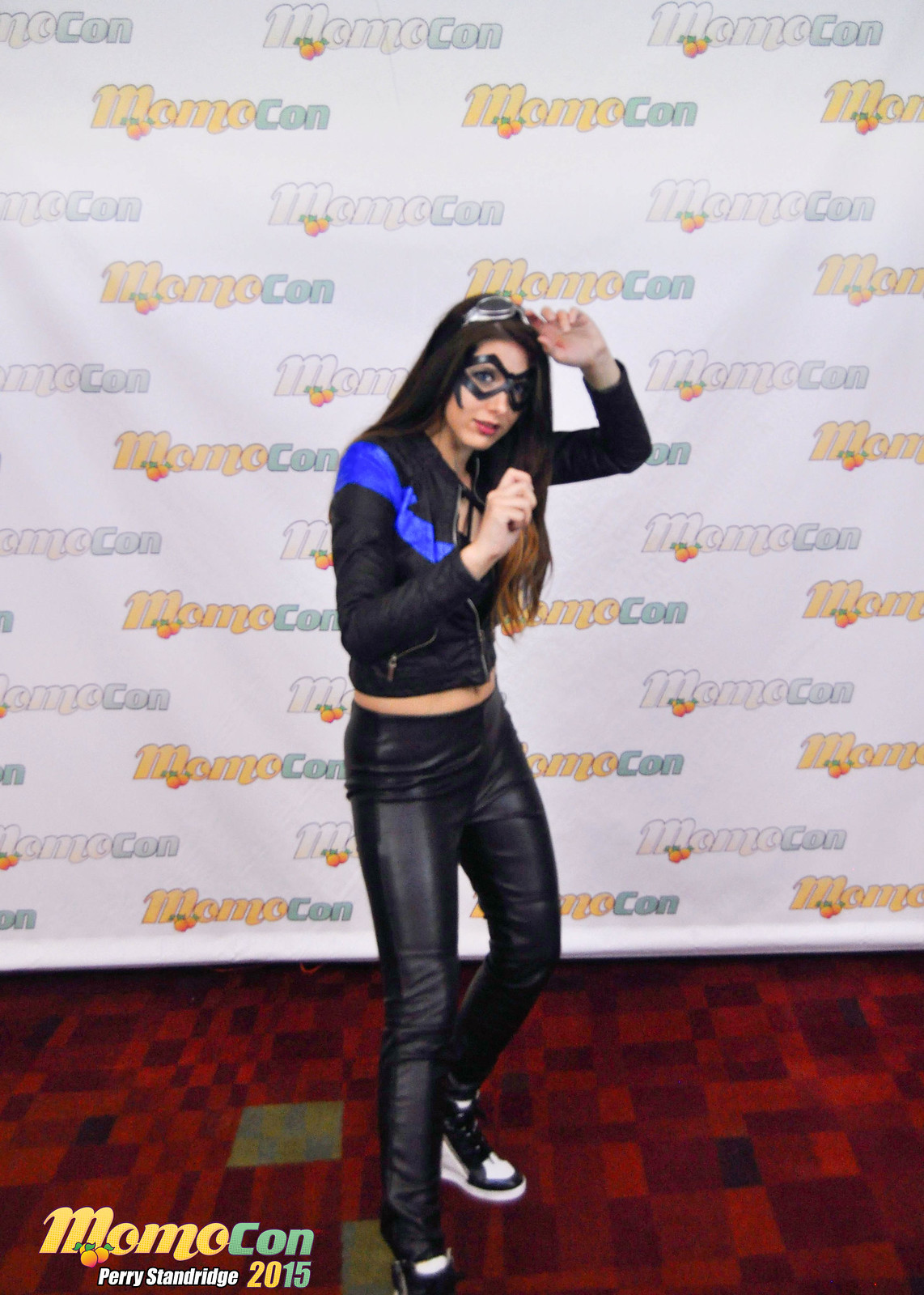The image captures a detailed color photograph of a young woman striking a martial arts pose at MOMOCON 2015. She stands confidently with her left hand raised to her forehead and her right hand positioned protectively near her chin. The woman has long dark hair with lighter brown tips and is adorned with red lipstick. She sports goggles on her head and a black domino mask that reveals her expressive eyes. 

Her attire consists of black leather pants and a trendy black and blue leather jacket with substantial zippers, partially unzipped to reveal her midriff. On her feet, she wears stylish black and white wedged sneakers. The backdrop is a white banner repeating the MOMOCON logo in various color combinations, flanked by a checkered black and red carpet underfoot. 

In the bottom-left corner of the image, the logo "MOMOCON" appears again, followed by the text "Perry Standridge, 2015" in white, marking the photographer and the year. This dynamic scene epitomizes the vibrant atmosphere of the convention, capturing not just a costume but an entire persona.